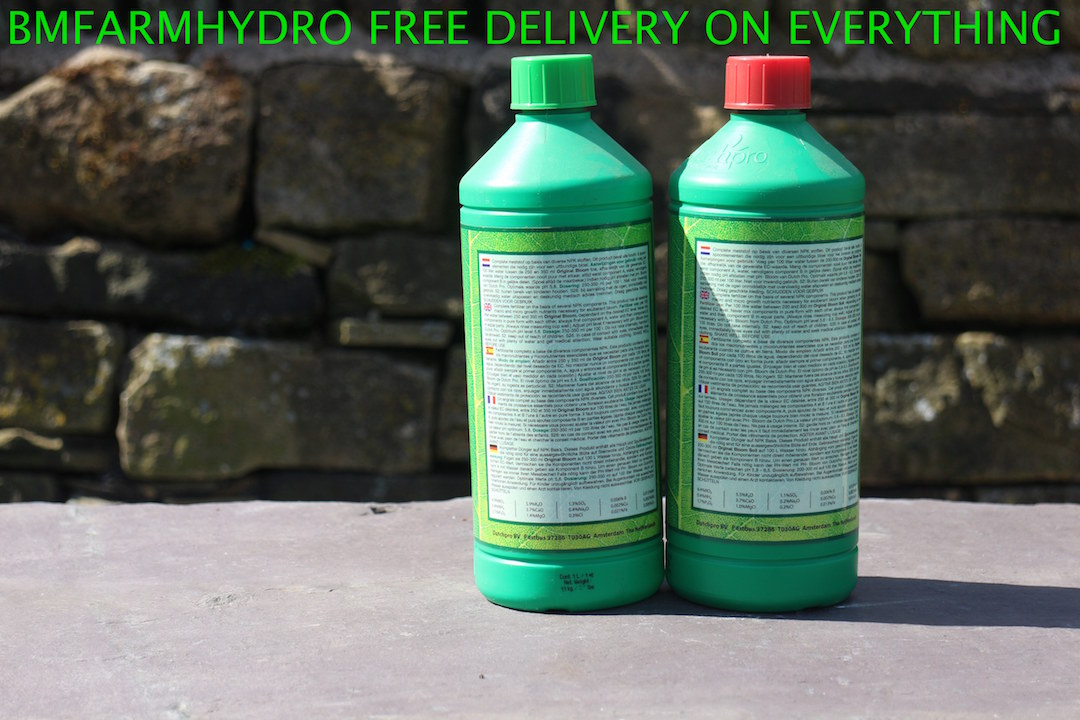This wide rectangular image showcases two quart-sized green plastic bottles, each adorned with distinctively colored caps—neon green for the bottle on the left and bright red for the bottle on the right. Both bottles feature a label bordered in a bright greenish-yellow, embellished with several tiny paragraphs of text, initiated by flags representing information in five different languages. Positioned just to the right of center, the bottles rest on a smooth gray rock surface, with a meticulously constructed stone wall of large misshapen grayish-green and brown bricks forming the backdrop. At the top of the image, a bold statement in neon green capital letters reads, "BM Farm Hydro, free delivery on everything," capturing attention and adding a commercial appeal to the scene.